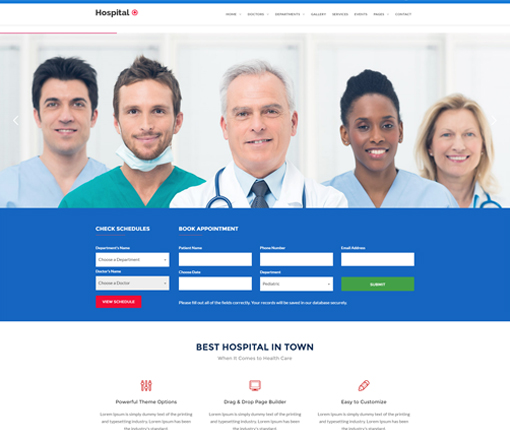The image appears to be a screenshot of a hospital's online portal. In the top left corner, the word "Hospital" is written in black text, accompanied by a red icon. Along the top edge of the screen, multiple grey tabs are visible, though the text on these tabs is largely unreadable due to the low resolution of the image.

Centrally featured is a photograph of five individuals. Positioned in the middle is an older gentleman wearing a white doctor's coat and a stethoscope, suggesting he is a physician. Flanking him are several individuals, some in blue and green scrubs, indicative of medical staff. On the left side of the image stands a woman also donned in a white medical outfit, likely another doctor. All appear to be smiling, and the photo captures them from the shoulders up.

Beneath the image is a blue section with the text "Check Schedules and Book Appointment". This area includes multiple white boxes, one of which is labeled "Choose a Department". Below these text fields is a green button labeled "Submit". In the lower left corner of this section, a red button labeled "View Schedule" is present.

At the bottom of the image, within a white strip, there is text that reads "Best Hospital in Town". This is followed by a message that states, "When it comes to healthcare", leading into three brief paragraphs. Each paragraph carries a different caption: "Powerful Theme Captions", "Theme Options", "Drag and Drop Page Builder", and "Easy to Customize".